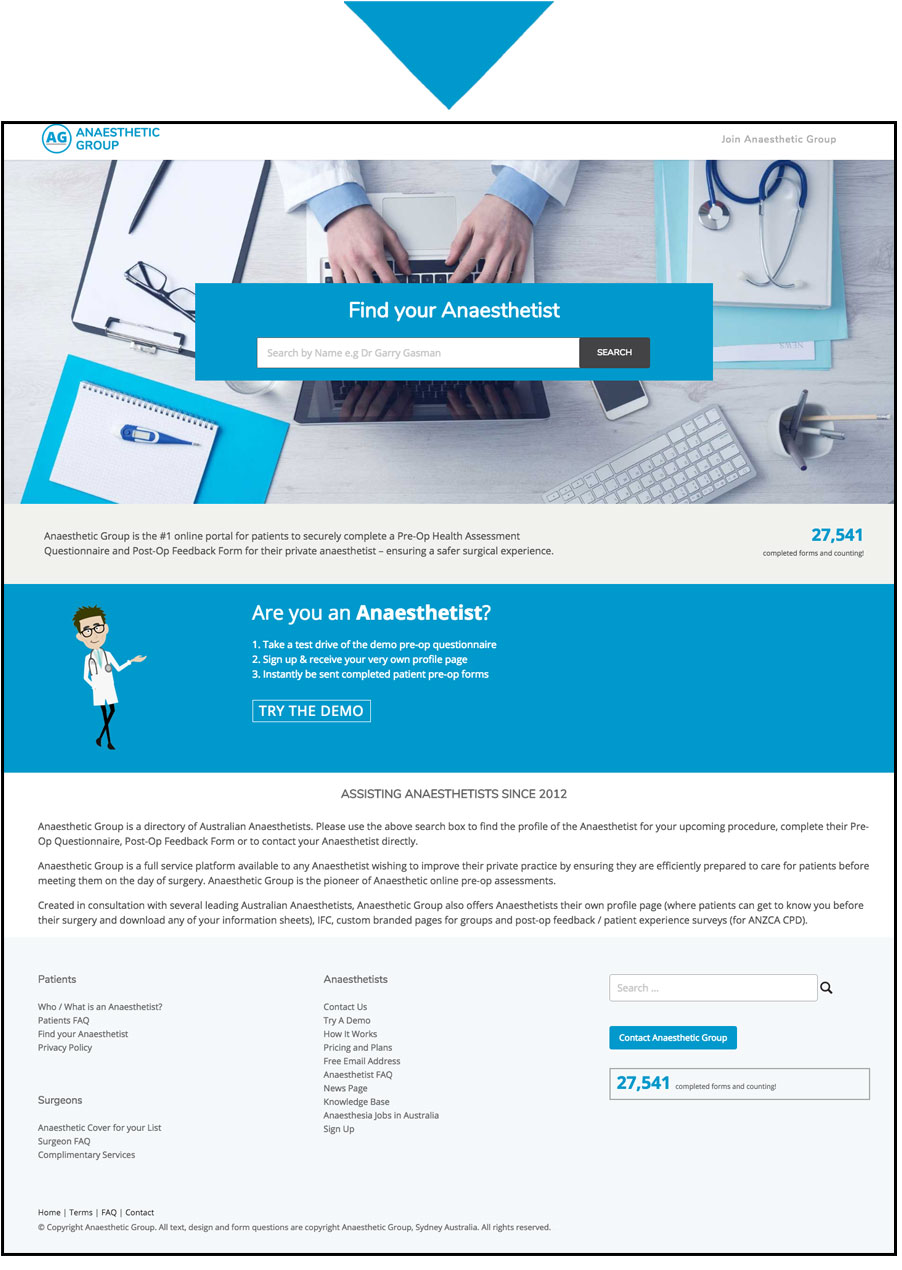The image appears to be a screenshot from a computer. At the top of the interface, there's a white section dominated by a large, inverted blue triangle. Below this, a white heading is displayed. In the upper left corner, the text reads "Anesthetic Group," accompanied by a circle containing the initials "AG."

Beneath this heading, an image spans the width of the screen, showing a doctor working on a laptop from a bird's-eye view, with only their hands visible. A blue pop-up window on the screen features the text "Find Your Anesthetist," alongside a search bar and a black search button.

Further down, there is more text, leading to a blue-bordered section that includes a cartoon graphic of a doctor. To the right of this graphic, promotional text reads, "Are you an anesthetist? Try the free demo."

At the bottom of the screen, a large gray rectangle contains the message, "Assisting anesthetists since 2012." This is followed by sections presumably containing information targeted at patients, surgeons, and anesthetists, repeated multiple times for emphasis.